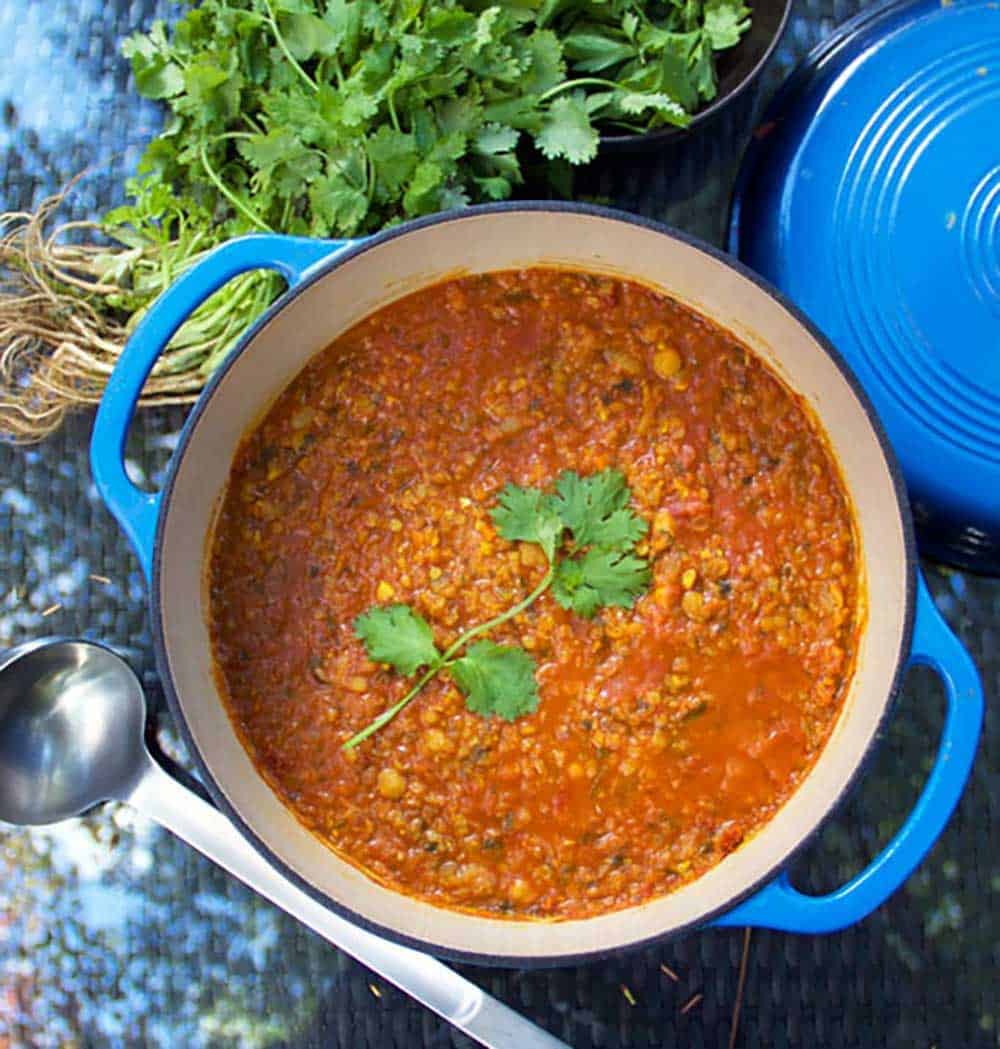The photograph captures a vibrant indoor kitchen scene centered around a hearty, red-orange stew that resembles chili. This thick, soupy stew, filling a white porcelain casserole dish with a blue exterior, is a medley of ingredients including corn kernels, black beans, grains, and larger lima beans. Crowning the dish is a decorative sprig of cilantro with four leaves. The casserole dish, featured prominently in the image, has handles facing the top left and bottom right corners. To the top left side of the dish, a matching blue lid, adorned with circles and ridges, rests slightly off-center. Scattered elements in the background include a black bowl brimming with green spices—possibly dill, cilantro, or parsley—positioned on a dark, multicolored table. This surface, displaying hues of dark brown, blue, gray, and red, is blurred, adding to the rustic ambiance. Completing the scene, a stainless steel ladle appears near the bottom right, suggesting readiness for serving this comforting and visually inviting meal.